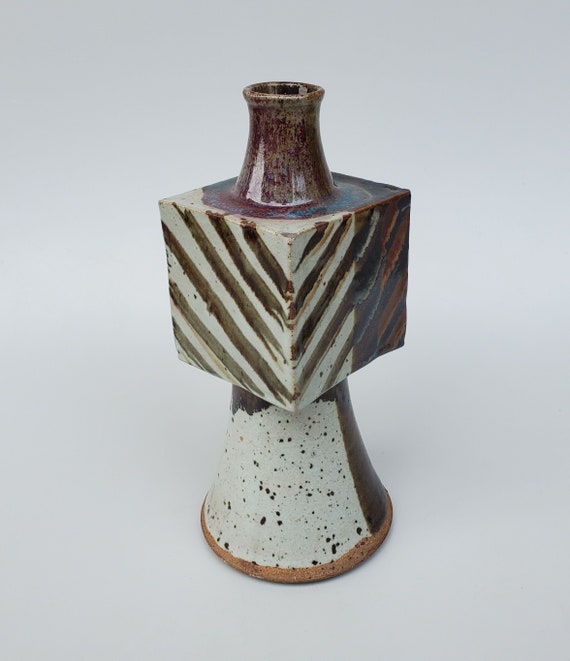This is a professional portrait photograph of an intriguing ceramic artwork set against a gray background. The piece is primarily a vase with a unique, multi-faceted design. At its core, the vase features a rugged, ancient look with 2-3 primary colors: tan, off-white, and a reddish-dark brown. The bottom of the vase is curved and tapers upwards, similar to the opening of a clarinet, and is particularly marked by a clear clay brown rim with black and white speckles.

Midway up the vase, a large, cube-like structure seamlessly intersects the cylindrical form. This tan square block displays intricate brown, red, and black angled stripes that extend towards its edges. Atop the block sits what resembles a shot glass with a bottle-like opening. The uppermost part of the vase is speckled white with black and transitions into a dirty maroon-brown hue.

Overall, this object stands as a striking vase formed by the melding of a cone and cube, displaying an exquisite blend of color and texture, with sharp diagonal angles meeting from two sides on the box section.